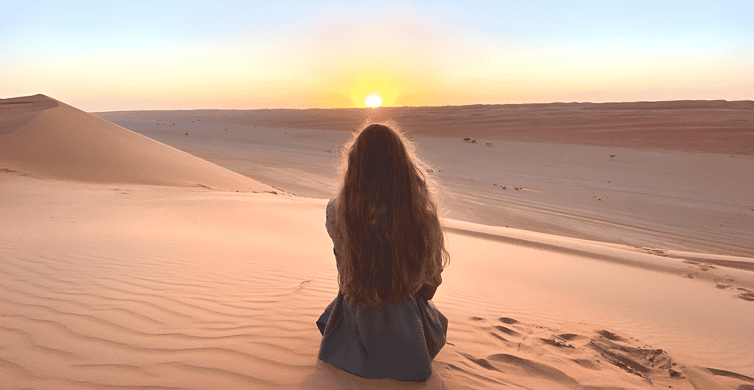In the image, a Caucasian woman with very long reddish-brown hair is seated on top of a vast sand dune, gazing out at a vibrant sunset on the horizon. Her back is turned to the camera, making her face unseen. The setting is a barren desert, characterized by endless waves of brown sand dunes stretching as far as the eye can see, devoid of any buildings or other people. She is dressed in a flowing dark blue robe, adding a touch of color against the endless monochrome of the desert landscape. The sky above is a mesmerizing palette, from deep oranges and yellows to washed-out blues, as the sun dips below the horizon.